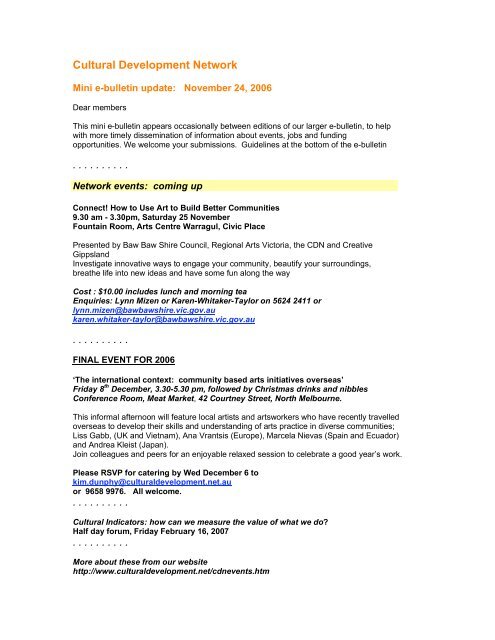The image captures a Cultural Development Network Mini-eBulletin Update dated November 24, 2006. This bulletin, occasionally issued between the larger eBulletins, aims to promptly disseminate information about various events, jobs, and funding opportunities. The bulletin is predominantly text-based, with a white background. "Cultural Development Network Mini-E-Bulletin Update, November 24th, 2006" is prominently displayed at the top in orange text, followed by a smaller black font addressing "Dear Members." Below this, a series of 10 dots create a border effect, separating different sections of the bulletin.

The first section, enclosed in a white rectangle border, highlights upcoming network events, providing details about the event time, location, presenters, costs, and clickable blue email addresses for further contact. Another dotted border separates this section from the "Final Event for 2006," which is emphasized with underlined and bolded text. This section similarly lists event details, including time, speakers, and email contacts. At the bottom of the bulletin, additional information appears about the organization's website and various forums and events scheduled, with a link to their webpage, http://www.culturaldevelopment.net.htm. The bulletin uses a range of colors including white, orange, light yellow, and blue to structure and highlight its content.